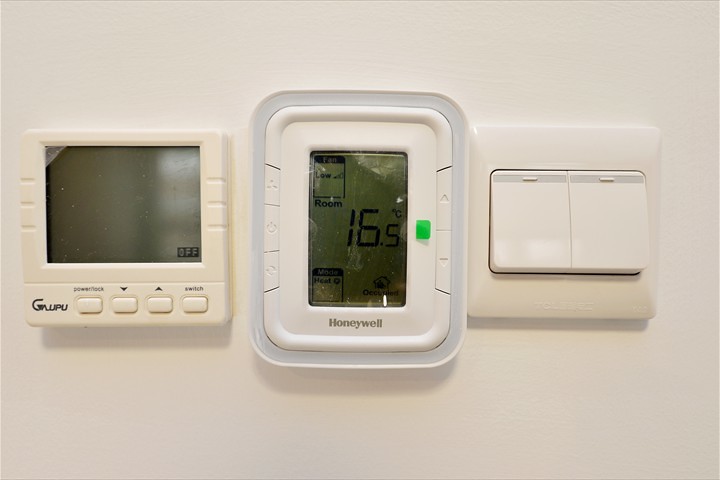In this landscape-oriented photograph, we see a close-up view of a white wall featuring three smart home controls. The central device is a Honeywell thermostat, distinctively taller than wide, which digitally displays a temperature setting of 16.5 degrees Celsius and indicates that the room is in "low mode." This thermostat, housed in white plastic, has a bright green light on the right side near the temperature display and includes several control buttons: a fan button, a power button, a recycle button, and two buttons for adjusting the temperature up or down.

Immediately to the right of the thermostat is a white light switch panel with two rocker switches in the 'up' position. To the left of the thermostat is an unidentified control device that is currently in "off" mode. This gadget, also encased in white plastic, features a digital screen and a series of labeled buttons at the bottom: "power and lock," a down arrow, an up arrow, and a switch button. The edges of the device are embellished with three decorative indents on each side. The bottom of this device is inscribed with the letters "GWPU," though its exact function remains unclear aside from its current off status.